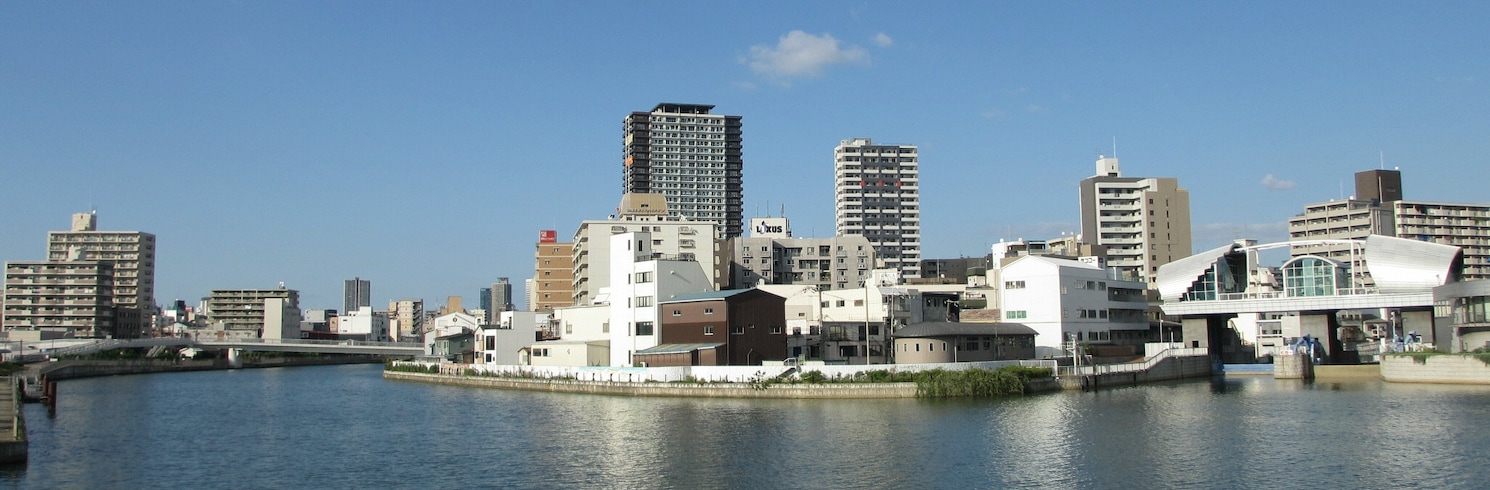The panoramic photograph captures a vibrant harbor city with a beautiful clear blue sky adorned by a single fluffy cloud. In the foreground, a wide curving river cuts through the urban landscape, flanked by a mix of high-rise and smaller residential buildings. The left side of the image features a straightforward driving bridge, while the right side showcases a more intricate bridge with a distinctive silver structure on top, possibly accommodating a tram or a pedestrian walkway connecting to significant buildings like a hospital. The water below is a calm, darkish blue, reflecting the tranquility of the scene. The city’s impressive skyline, dotted with several tall skyscrapers, towers above an array of smaller white buildings, completing this breathtaking daytime view of the metropolitan harbor.